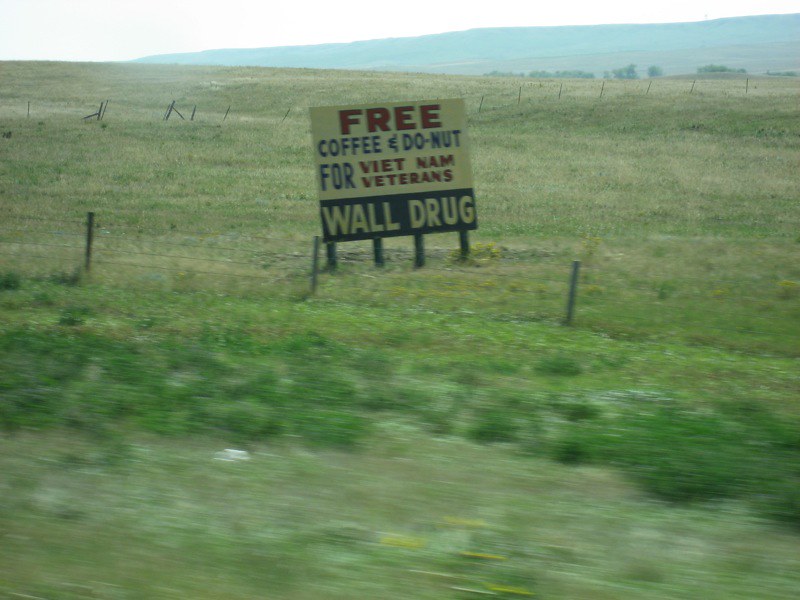The photo captures a moment from inside a moving vehicle, revealing a vast landscape predominantly composed of green and brownish-yellow fields, indicating a combination of lush and dry grass. The foreground is slightly blurry, emphasizing the motion of the car. In the middle of this expansive land, a prominent sign supported by four wooden posts takes center stage. The sign is segmented with "FREE" written in bold red letters, "COFFEE AND DONUTS FOR" in blue, "VIETNAM VETERANS" again in red, and "WALL DRUG" written in white on a blue background. Visibility is further enhanced by a white border around the main message and a blue ribbon-like design. The scene also includes a fence made of wire held by three wooden beams to restrict access, with trees and a hill visible in the background, completing the countryside vista.